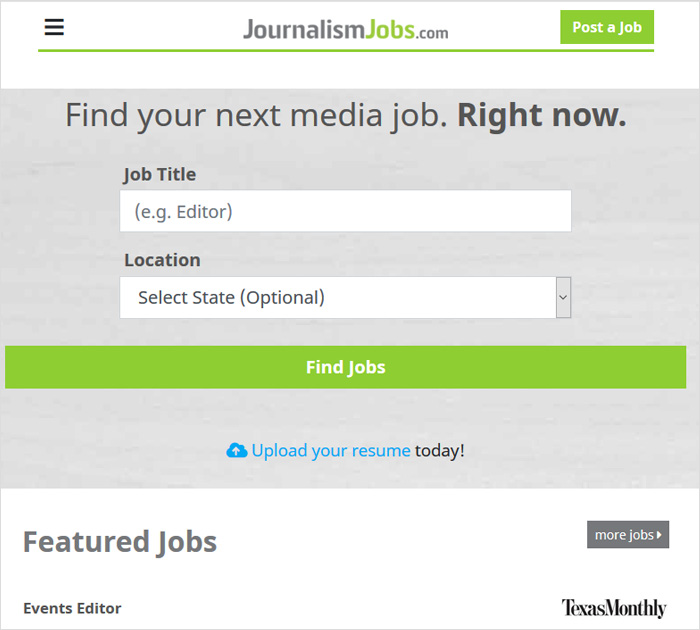The image depicts a clean and straightforward user interface for JournalismJobs.com. At the top center of the display, the site's name is prominently featured with "Journalism" in gray and "Jobs" in vibrant lime green, followed by ".com" in black. To the right, there is a matching lime green button labeled "Post a Job."

Set against a simple gray background, the main header reads "Find Your Next Media Job" in bold black text. Below this, there are input fields for users to type in a job title, such as "Editor," and an optional location selector with a dropdown menu labeled "Select State."

Spanning the entire width of the page is a lime green bar with the text "Find Jobs." Just beneath this, a blue cloud-shaped button invites users to "Upload Your Resume," with the word "Today" in gray.

Further down, in larger lettering, the section titled "Featured Jobs" is displayed. To the right of this section is a clickable box that says "More Jobs." Finally, in the bottom right-hand corner, there is a mention of "Texas Monthly," posted by the Events Editor.